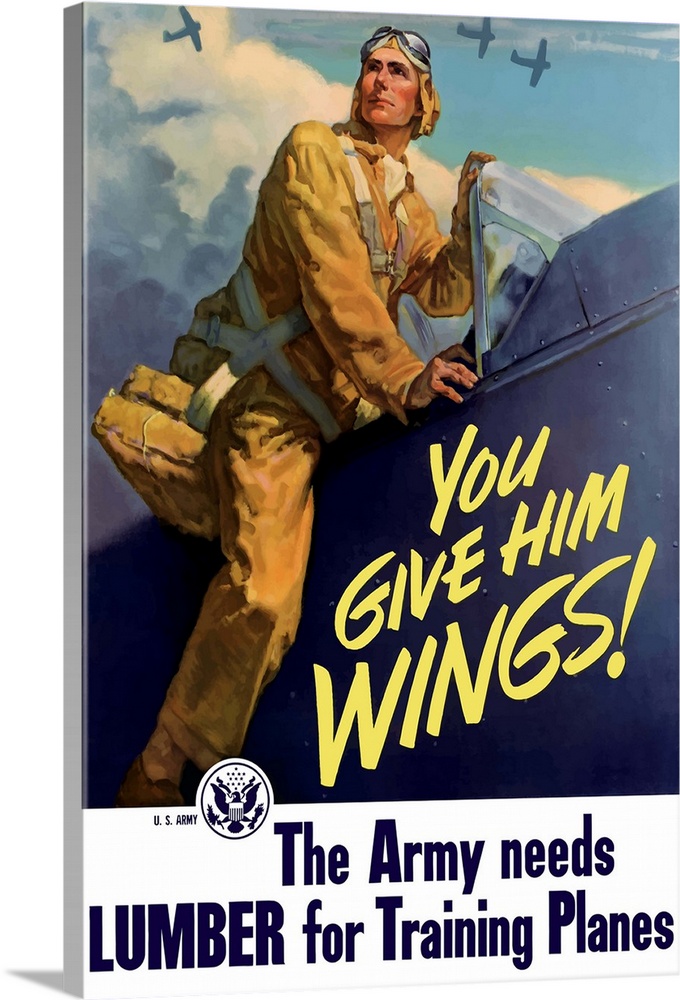This World War II-era poster serves as an advertisement for the U.S. Army, emphasizing the message "The Army needs lumber for training planes." Prominently featured is a determined-looking man wearing a tan pilot suit, goggles, and a pilot hat, with a parachute attached to his back, as he steps into the open cockpit of a blue aircraft. On the side of the plane, in bold yellow text, it states "You give him WINGS." Above this text, there is an elaborate depiction of the U.S. Army insignia. In the background, three fighter planes can be seen soaring through the cloudy sky, potentially engaged in a training exercise or dogfight, underscoring the urgency and bravery of the pilots. This evocative imagery is crafted to rally civilian support, encouraging them to supply the necessary lumber to build training planes, thus bolstering the war effort.